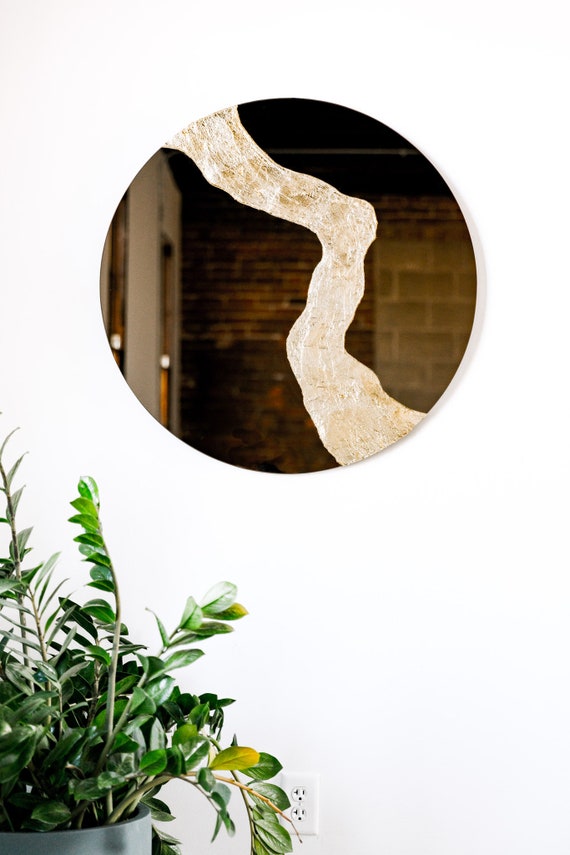The image features a clean and simple white wall with a power outlet positioned near the bottom. To the left, the top of a gray pot is visible, housing a lush green house plant with long stems and small green leaves. Prominently centered on the wall is a round mirror with a minimalist white frame. The reflection in the mirror captures an intriguing, abstract scene: an irregular, tube-like shape reminiscent of a tree trunk or a piece of web, set against a backdrop of a brick wall. Visible in the mirror's reflection are architectural elements including a doorway on the left and possibly additional doorways, with some white lights appearing blurry in the background. A faint gray shadow subtly outlines the circular mirror, adding to the visual depth of the setting.